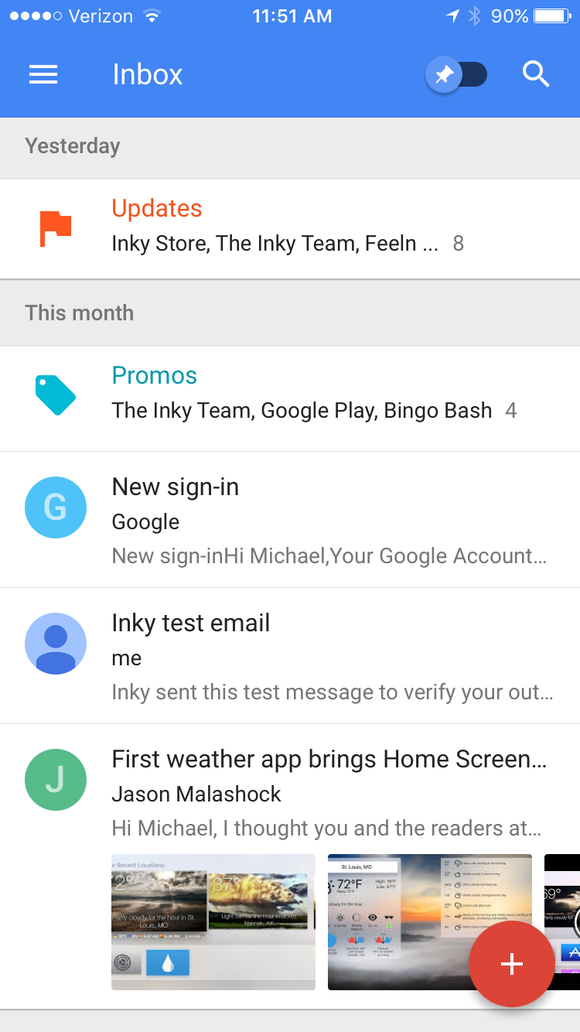Screenshot of an email inbox with a blue-themed interface. The top of the inbox displays the label "Yesterday." The first message is an "Update" from the Inky Store, highlighted with a mix of black and red text. It indicates there are eight new messages in total.

Below, a section titled "This Month" categorizes emails under various tags. One tag, labeled "Promos" and colored teal, sorts promotional emails. The messages under this tag include notifications from "The Inky Team," "Google Play," and "Bingle Bash" with four related emails. 

A security alert email indicates a "New sign-in on Google" titled "Michael, your Google account." Additionally, there's a test email from Inky stating, "Inky sent this test message to verify your..." with the rest of the message truncated.

Also featured is an email from a sender identified as "J," with a green background, discussing a new update, titled "First weather app brings home screen." The sender, Jason Malishock, starts the message with, "Hi, Michael. I thought you had the readers at...," trailing off.

There are three image attachments displayed at the bottom of the screenshot.

In summary, the descriptive snapshot highlights the user's inbox layout, categorized tags, email sources, and the specific content of select messages.